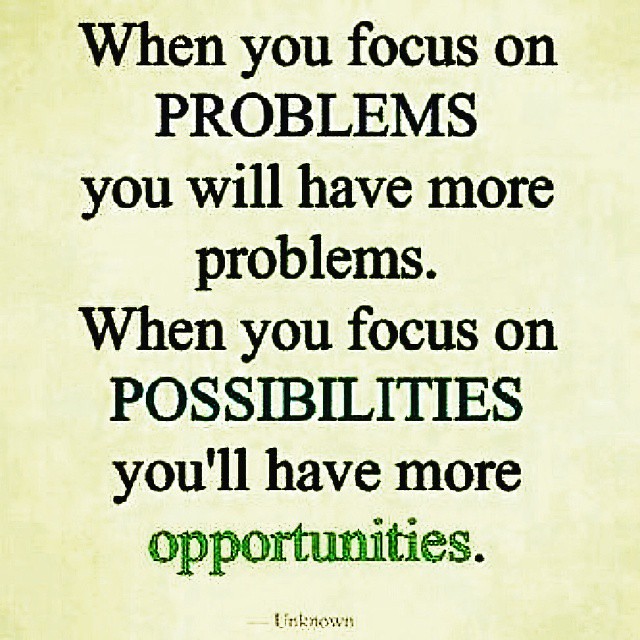The image is of a quote with a high-contrast text arranged center-aligned on a background that transitions from a light brown to a cream shade, creating a gradient effect that highlights the text. The background, though somewhat artifacted and blurry in parts, fluctuates in shade, making the words stand out more sharply in focus. The quote reads, "When you focus on problems, you will have more problems. When you focus on possibilities, you'll have more opportunities." The words "PROBLEMS" and "POSSIBILITIES" are distinctly capitalized to draw attention. The word "OPPORTUNITIES" is uniquely colored in green, contrasting with the otherwise black text. At the very bottom, in smaller font, the word "unknown" is written in the center, providing the attribution.